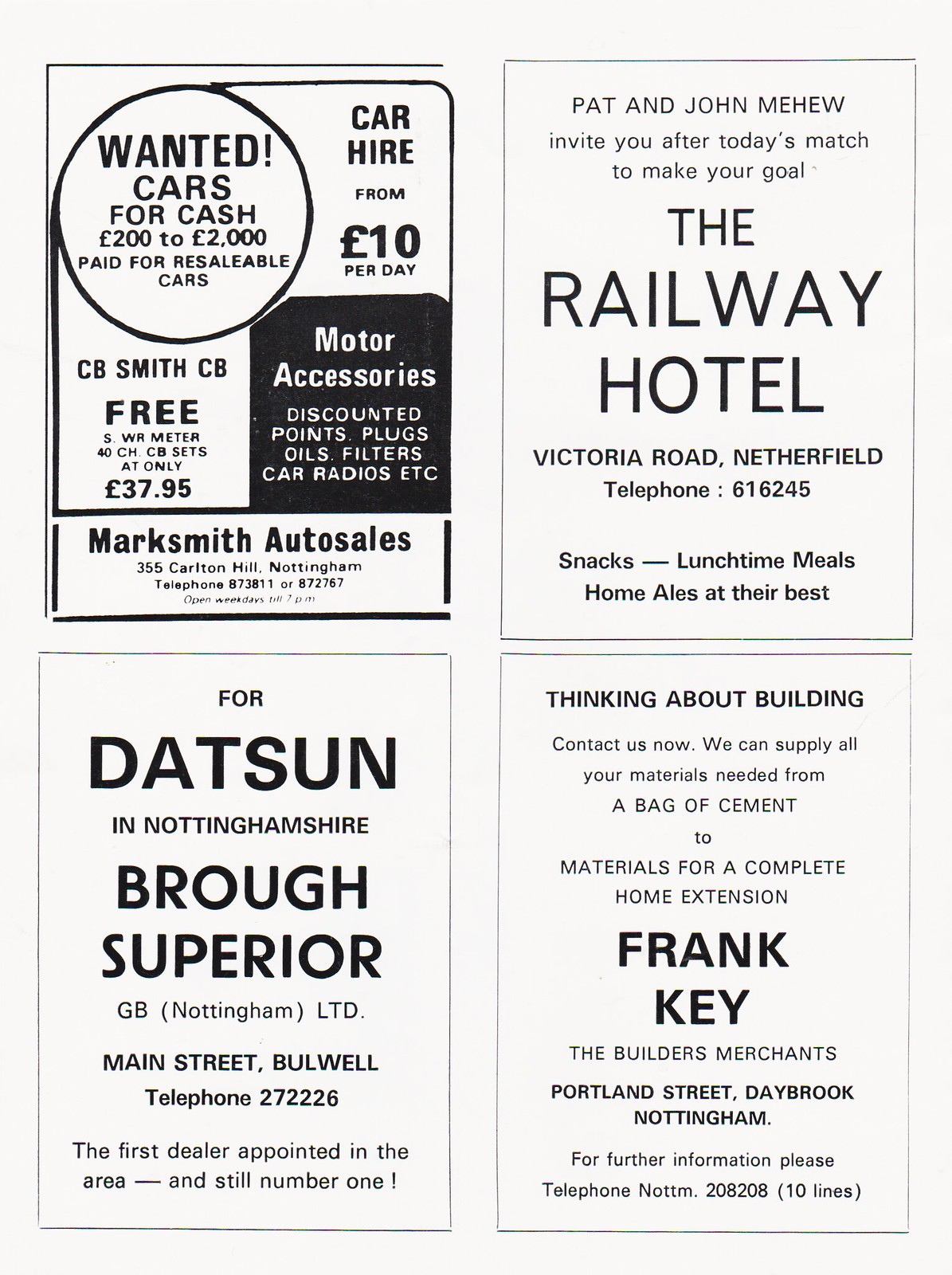The image displays a page divided into four equal rectangular advertisements arranged in two columns. 

1. The top left ad, for Mark Smith Auto Sales, features various offers including "Wanted: Cars for Cash," paying between 200 to 2,000 pounds for resaleable cars, and car hire starting at 10 pounds per day. Additionally, it mentions several motor accessories and provides the address, 355 Carlton Hill, Nottingham, and their contact numbers, with detailed hours of operation.

2. The top right ad is an invitation from Pat and John Mayhew encouraging viewers to visit the Railway Hotel on Victoria Road, Netherfield, after today's match. The ad highlights the availability of snacks, lunchtime meals, and high-quality home ales. The contact telephone number provided is 616-245-SNACKS.

3. The bottom left ad promotes Ford Dotson in Nottingham and Brough Superior, operated by GB Nottingham LTD on Main Street, Bullwell. It boasts being the first dealer appointed in the area and remains number one, with a contact number of 272-226.

4. The bottom right ad is for Frank Key, the builder's merchant located on Portland Street, Daybrook, Nottingham. It invites potential customers who are considering building or extending their homes to contact them for all necessary materials, from bags of cement to complete home extension supplies. For further inquiries, the telephone number provided is Nottingham 208-208, with 10 available lines.

Together, these ads create a vivid depiction of various services available in Nottingham, from auto sales and hotels to construction supplies.